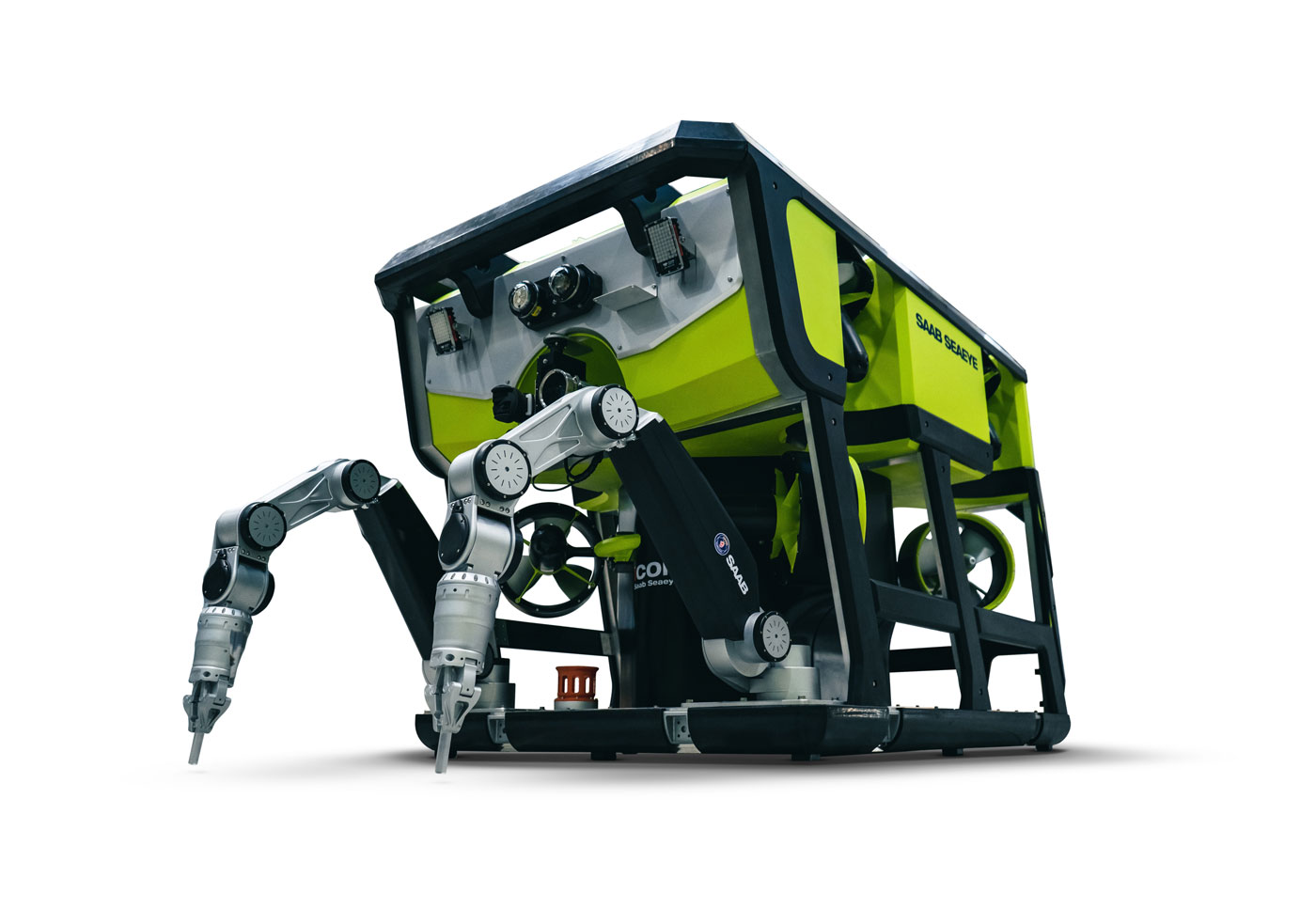The image displays a modern and sophisticated robotic machine, primarily square in shape, positioned against a white background that accentuates its features. The robot has a combination of green and black colors, with accents in yellow, silver, and gray. It features two metal robotic arms extending from its back, which have small black fan-like components on either end. 

Text on the robot includes the difficult-to-read words "Saab Sears" on its side and "GAAB" on one of the arms. There's also a red object attached to the bottom of the machine, possibly a functional component. The machine's design includes front elements that might be cameras or lights, suggesting it could be used for navigation or surveillance in environments inaccessible to humans. Shadows on the floor enhance the aesthetic, making the image appear as a product advertisement showcasing this advanced robotic technology, potentially for use on land, water, or tight spaces.